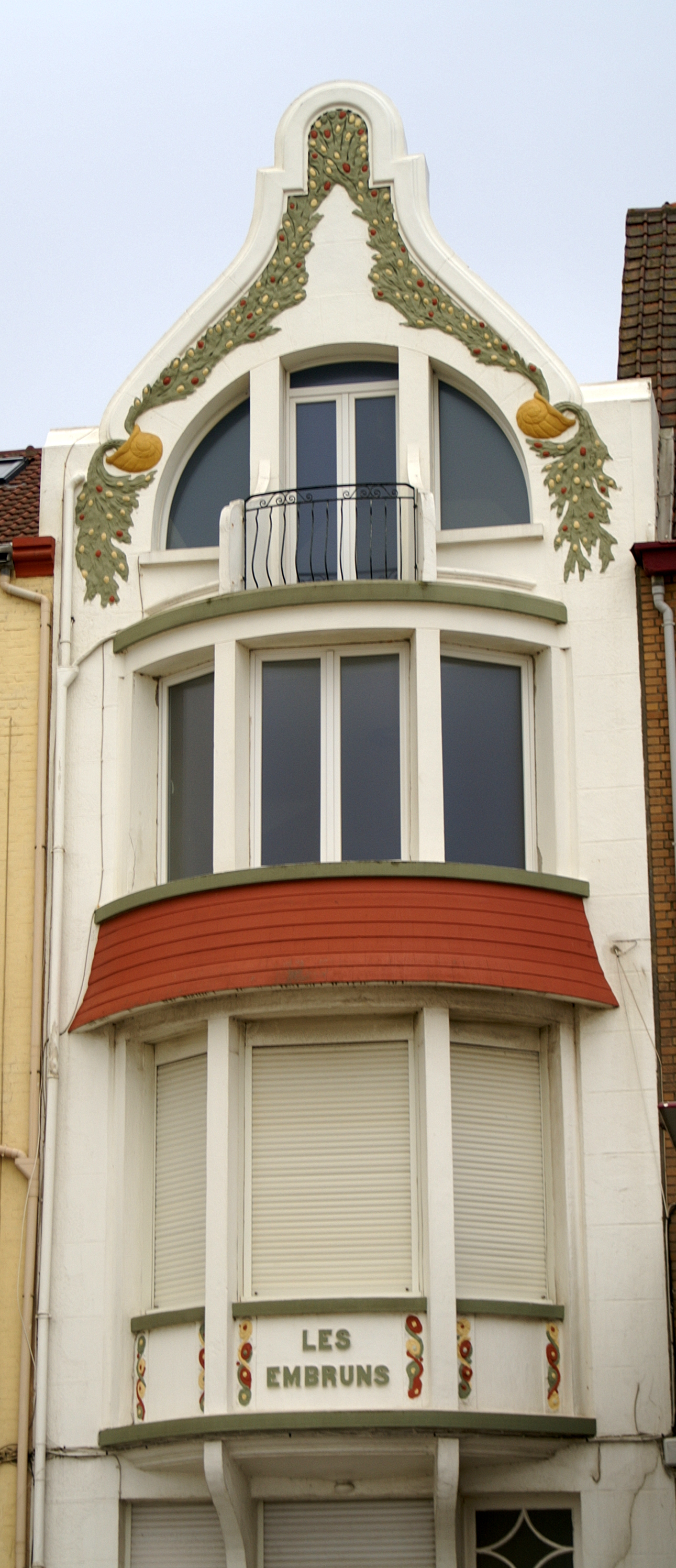This highly detailed photographic image captures the front facade of a narrow, three-story building nestled between two other structures, set outdoors during the daytime under a clear blue sky. The building stands out with its distinct architectural elements that evoke an old-world charm reminiscent of Cuban or Latin American aesthetics. At the very top, the building features an arched roof, ornately decorated with permanent green leaves and golden helmet-like embellishments. A prominent arched window is situated just below this decorative top.

The second story showcases a small balcony with a black metal railing, accessible via two rectangular doors. Below this balcony is a series of four narrow, darker windows, reinforcing the building’s vertical elegance. The entire structure is painted in pristine white, except for a contrasting red brick or stucco ledge directly below the second story windows.

The ground level is marked by three wider windows and a notable red awning that curves outward, adding a splash of vibrant color to the scene. Prominently displayed beneath the awning is a sign reading “Les Embruns.” The base of the building also features a small window and hints at what may be an entryway or the start of a doorway. The building's overall architectural detailing, the color contrasts, and the intricate design elements make it a striking and picturesque edifice.